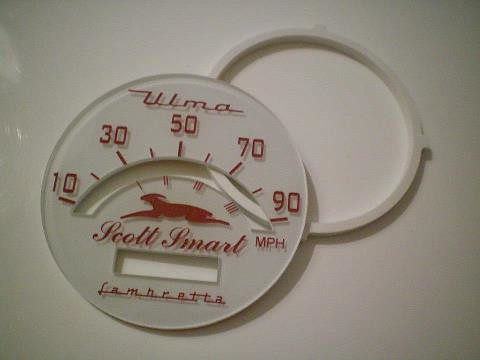The image showcases a speedometer gauge set against a pristine white background. The background features a subtle grayish tint with occasional white paint spots visible, particularly on the left-hand side near the top of the image. The gauge itself is mounted on a white rubber gasket that has small evenly-spaced studs around the perimeter, visible on the top, right, and bottom edges (the left side is obscured). The gauge is encased in what appears to be a frosted or semi-opaque glass finish, giving it a sleek and polished look.

In the center of the gauge’s face, it is adorned with the words "Got Smart" and an image of a running deer, both rendered in red. Above the display, the acronym "ULMA" is prominently displayed in matching red text. The speed markings on the gauge are also in red, starting from 10 MPH on the left and increasing incrementally by 20, up to 90 MPH on the right. At the bottom of the gauge, the brand name "Lambretta" is distinctly written in red text, completing the intricate and detailed design of this vintage-inspired speedometer.